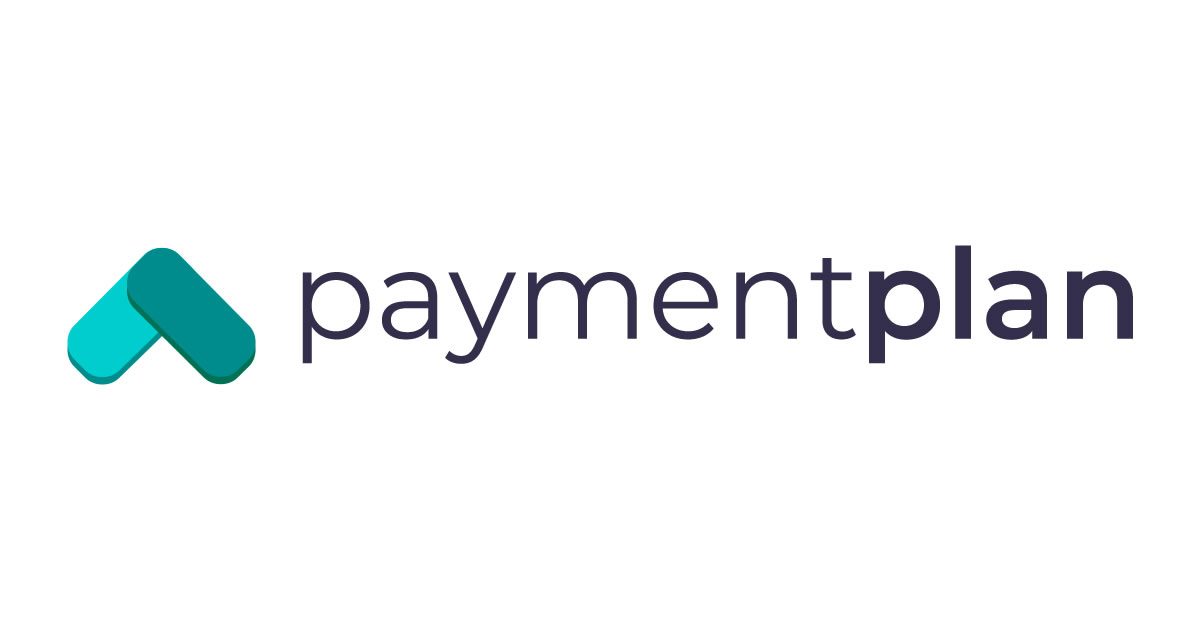The image showcases a clean and minimalist logo for an entity, perhaps related to financial services or digital solutions. It features a solid white background, providing a stark contrast to the elements on it. On the left side of the image, there is a logo consisting of two teal rectangles with rounded edges, positioned at a diagonal 45-degree angle. The rectangle on the left is a lighter shade of teal, pointing its top toward the right, while the rectangle on the right is a darker shade of teal, with its top angled toward the left. These shapes converge at their top edges, creating a unified, dynamic look.

To the right of the logo, the word "paymentplan" is written in a font so dark navy blue that it appears almost black. This text is highly rounded, contributing to a friendly and approachable appearance. Notably, the word "payment" is presented in a regular weight, whereas "plan" is emphasized with bold lettering. This typographic distinction subtly highlights the planning aspect of the service or product being offered. The entire composition is clear and concise, making it easily recognizable and memorable.